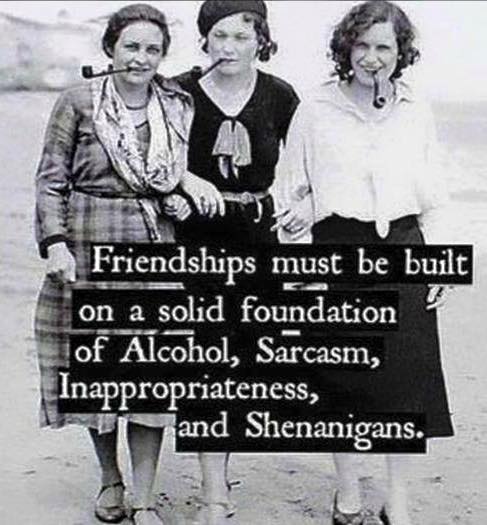In this black and white image, three women stand together on a beach, their arms interlocked in a moment of camaraderie. Each woman has a smoking pipe in her mouth, adding a touch of rebellion to their elegant poses. They are dressed in long dresses and wearing sandals, standing on sand. The woman on the left wears a flannel plaid dress with a large scarf around her neck, and her hair is pulled back. The woman in the middle, distinguishable by her all-black dress with tassels around the bosom and a dark hat, has her eyes closed. The woman on the right sports a white button-down shirt with a long black skirt, her shoulder-length curly hair framing her face. Across the middle of the image, the text reads: "Friendship must be built on a solid foundation of alcohol, sarcasm, inappropriateness, and shenanigans." This classic scene, with its shades of blacks, whites, and grays, captures the timeless essence of strong, spirited friendship.